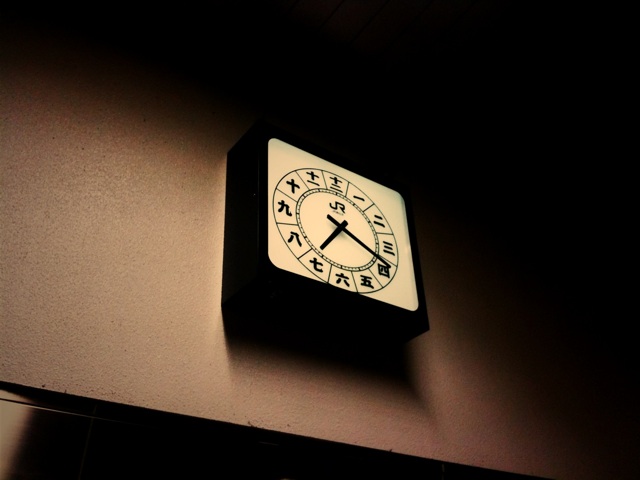This image features a black wall clock with a white face, set against a gray background. The clock face is adorned with what appear to be Asian characters, though their specific language is unidentifiable. The clock's hands are positioned at what would be the equivalent of 4:20. The design incorporates a short hour hand and a long minute hand. Notably, the clock includes a variety of symbols, such as a cross, a cross with a line underneath it, a cross with two lines below, as well as symbols representing single, double, and triple lines. Additionally, there are markings resembling a small square, a T, and a lowercase "r." At the bottom of the clock, a black shadow is cast, emphasizing the depth of the clock housing, which extends a few inches outward from the background.